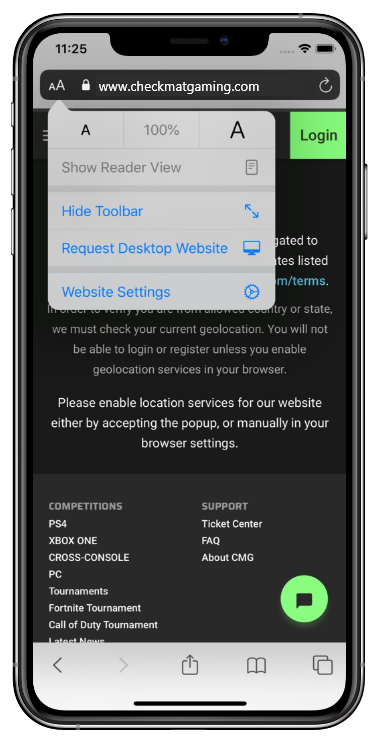This image is a detailed screenshot showing a phone in its entirety, including the full sleek silver casing with clearly visible side buttons. The power button is positioned on the upper right side of the phone while the volume buttons are located on the upper left. The screen displays a website, checkmatgaming.com, with the browser's address bar at the top. To the left of the URL, the time reads 11:25, and to the right, the battery icon is displayed. Adjacent to the address, there is a drop-down window linked to the 'AA' icon, providing options such as 'Hide Toolbar,' 'Request Desktop Website,' and 'Website Settings,' all highlighted in blue.

The webpage itself features a black background with a green 'Login' button under the address bar. The visible text, although partially obscured by the pop-up window, includes a message near the bottom requesting users to enable location services for the website, either via a pop-up or manually through browser settings. Below this instruction, there's a small dark grey chart divided into two sections: 'Competitions,' which lists multiple items, and 'Support,' with a shorter three-item list. In the bottom right corner of the screen, a green message button is noticeable. The phone’s footer includes three icons, among them a bookmark icon and an upload icon, enhancing navigational ease.